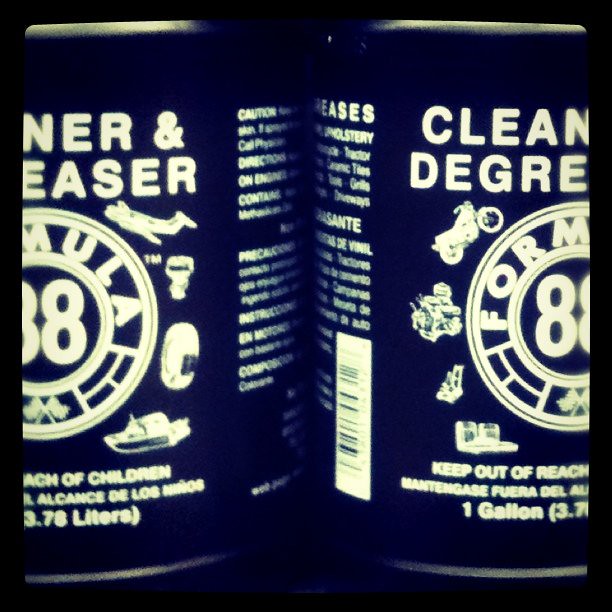This vibrant close-up photograph showcases two large cylindrical dark green cans of cleaner and degreaser, partially visible due to their cropped edges. Clearly labeled with various designs, both cans feature a prominent round logo, each bearing a number 8 within a circle. The logo is surrounded by flags and partially legible text, with discernible images of an airplane, a motorcycle, and other equipment such as a tire and a ship, indicating the multi-purpose utility of the solutions. The Spanish phrase "Alcalance de los Niños" and the English phrase "Keep out of reach of children" are visible near the bottom, highlighting safety instructions. The cans are marked to have a capacity of one gallon, displayed as "3.8 liters" and "3.7 liters" respectively. The background text includes additional cautionary measures, emphasizing the need for careful handling of the product. The photograph's meticulous details bring out the caution and utility of the cleaning solution contained within the cans.